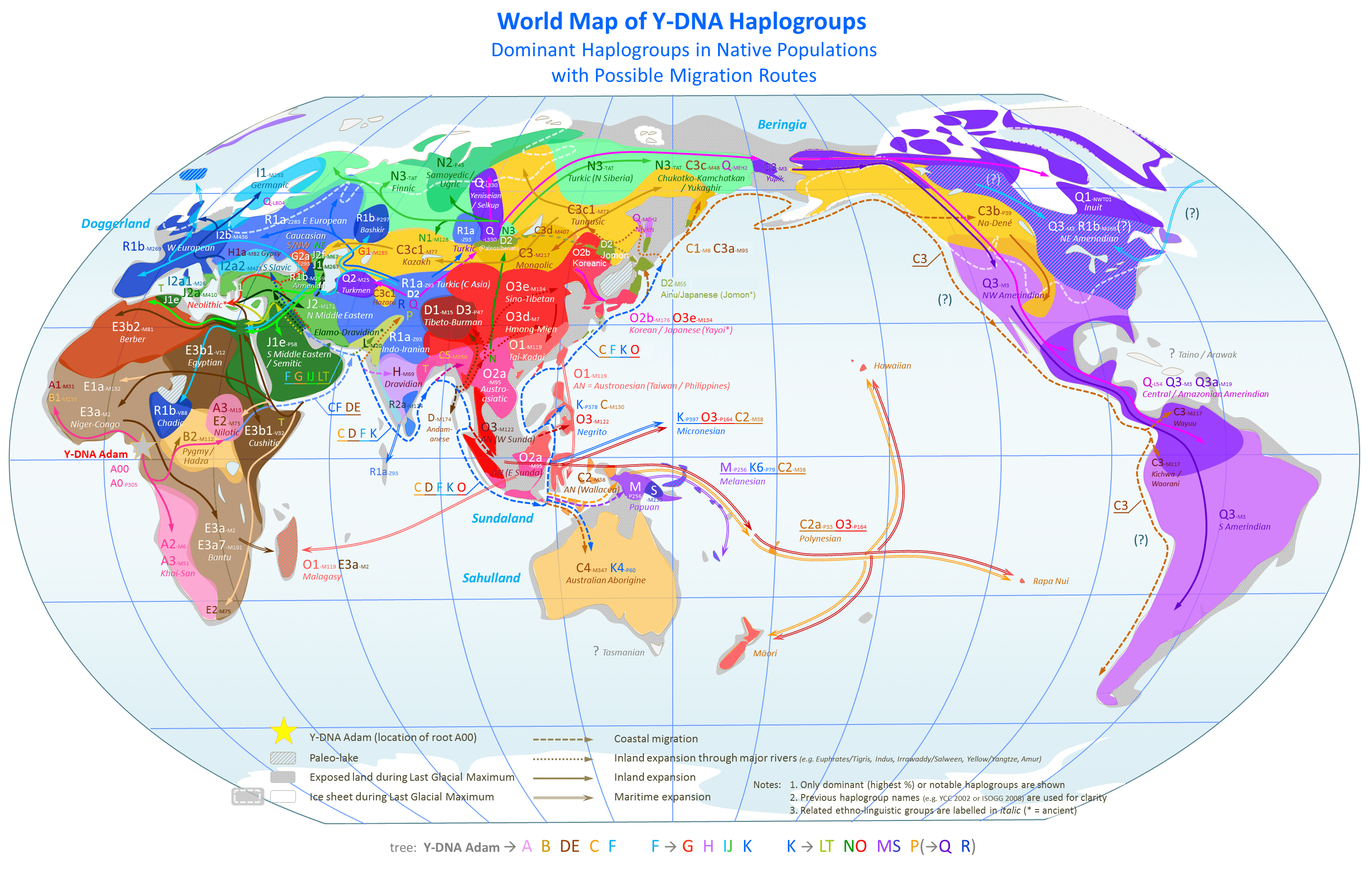This vibrant, detailed world map, titled "World Map of Y-DNA Haplogroups," illustrates the dominant Y-DNA haplogroups among native populations, including possible migration routes. Unlike traditional maps, this map situates North America and South America to the far right, placing a greater emphasis on Europe, Asia, and Australia, which occupy the central section. Color-coded regions vividly represent various haplogroups across continents, except for Antarctica, which remains uncolored and stark white. Intricate arrows trace historical migration routes, providing a glimpse into human movement patterns. The United States predominantly features shades of purple and periwinkle interspersed with patches of yellow. Additionally, the map showcases a variety of symbols and scales, including a prominent yellow star and numerous gray areas, enhancing its complexity and informational depth. The vast oceanic regions are clearly depicted, framing the multi-hued continents and reflecting the global focus of this genetic map.